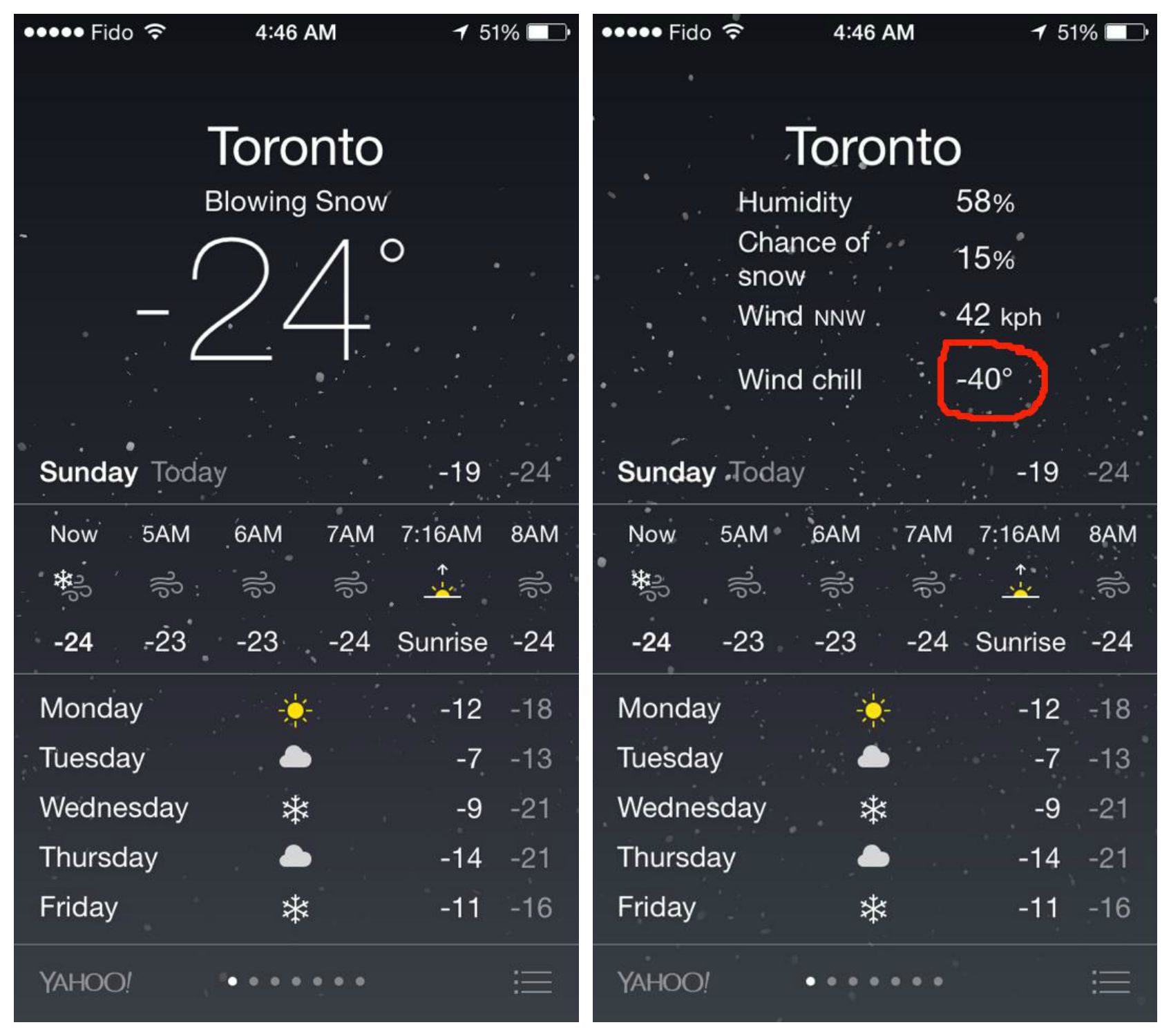The image showcases a detailed depiction of weather information from two smartphone screenshots in portrait format. Both screenshots display weather data with the following layout:

### Left Screenshot:
- **Header:**
  - **Carrier:** "Fido" in white text, accompanied by five white dots and a white reception bar icon.
  - **Time:** "4:46 a.m."
  - **Battery:** "51%" with a white battery icon.
- **City:** "Toronto"
- **Weather:**
  - **Condition:** "Blowing snow"
  - **Temperature:** "-24°C"
- **Additional Information:**
  - **Day/Date:** "Sunday"
  - **Today’s Forecast:** High of "-19°C" and low of "-24°C"
  - **Time Range:** Displays weather from the current time until 8 a.m., including a graphic of a gust of wind with a snowflake.
  - **Sunrise:** "7:16 a.m."
  - **Weekday Forecast:** Icons and temperatures for Monday through Friday, including images of a sun, a cloud, and a snowflake.

### Right Screenshot:
- **Header:**
  - **Carrier:** Same as the left screenshot.
  - **Time:** "4:46 a.m."
  - **Battery:** "51%"
- **City:** "Toronto"
- **Weather:**
  - **Humidity:** "58%"
  - **Chance of Snow:** "15%"
- **Wind:**
  - **Direction:** "North-Northwest"
  - **Speed:** "42 kilometers per hour"
  - **Wind Chill:** "-40°C" marked with a red circle for emphasis.

This visually rich and highly detailed caption captures the essence and nuances of the weather data displayed on both smartphones.